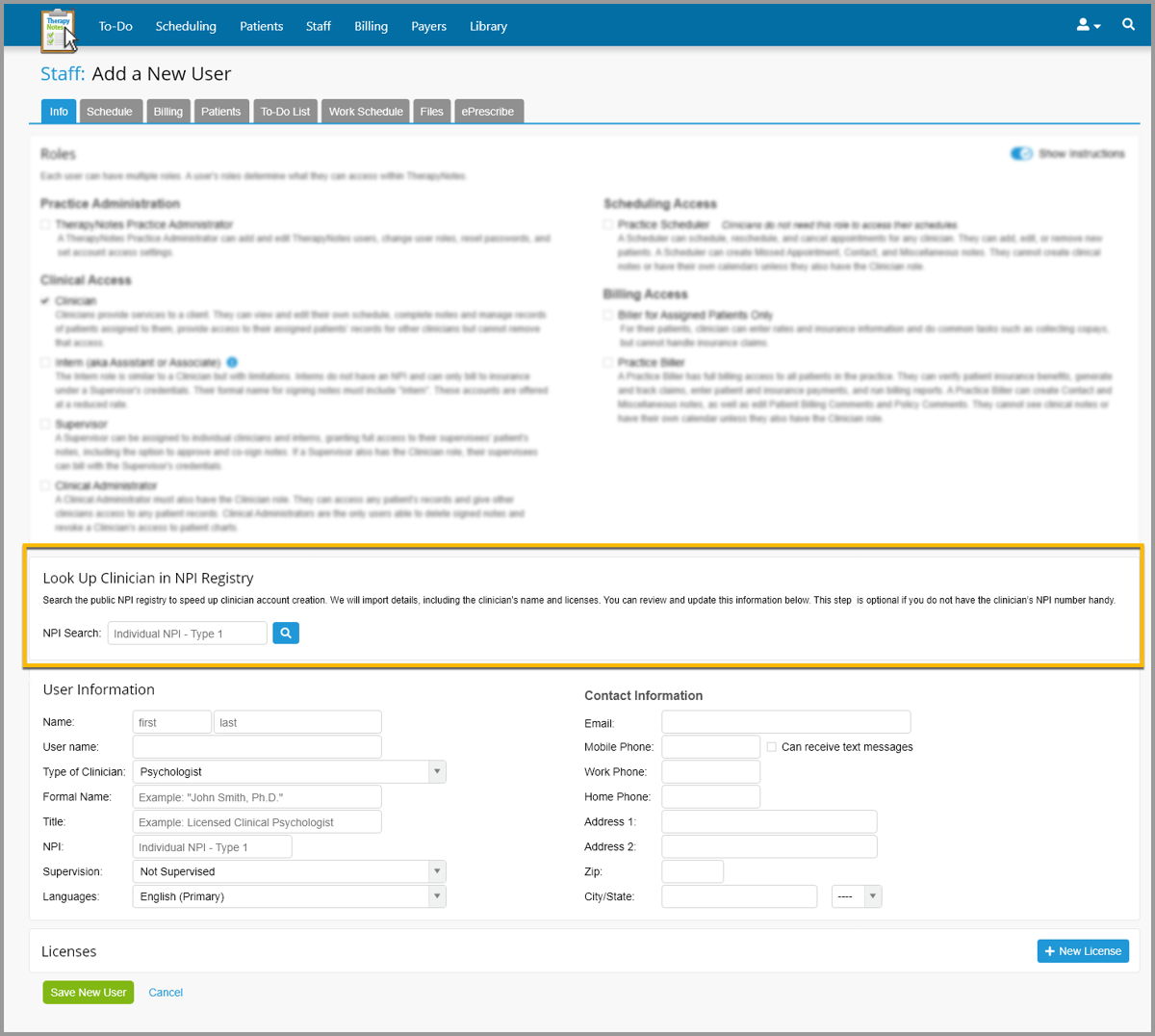The image showcases a screenshot from a medical practice management software interface. At the top of the screen, there is a blue bar featuring a logo of a clipboard with writing on it and a pointer directed at the clipboard. This is followed by a standard navigation bar with options for scheduling, patients, staff, billing, payers, and library. The staff page is currently selected, as evidenced by the "Staff: Add a New User" heading below the navigation bar.

The interface utilizes a tabbed layout, including tabs labeled Intro, Schedule, Billing, Patients, To-do List, and Work Schedule, although two of the tabs are unclear. The section below the tabs contains somewhat blurred text, displaying categories such as Practice Administration, Clinical Access, Scheduling Access, and Billing Access. These categories appear to be settings or permissions for the new staff member.

Further down, outlined in a yellow box, is a section titled "Look up Clinician in NPI Registry." This section allows users to search the public NPI (National Provider Identifier) registry to expedite clinician account creation. The software offers to import details—such as the clinician's name and licenses—for review and updates. This step is optional if the clinician's NPI number is not readily available.

The final part of the screen includes a searchable field for entering the clinician’s NPI number. Below this, there is a "User Information" form to fill out details like the clinician's name, type and formal title, NPI number, supervision details, languages spoken, and additional contact information.